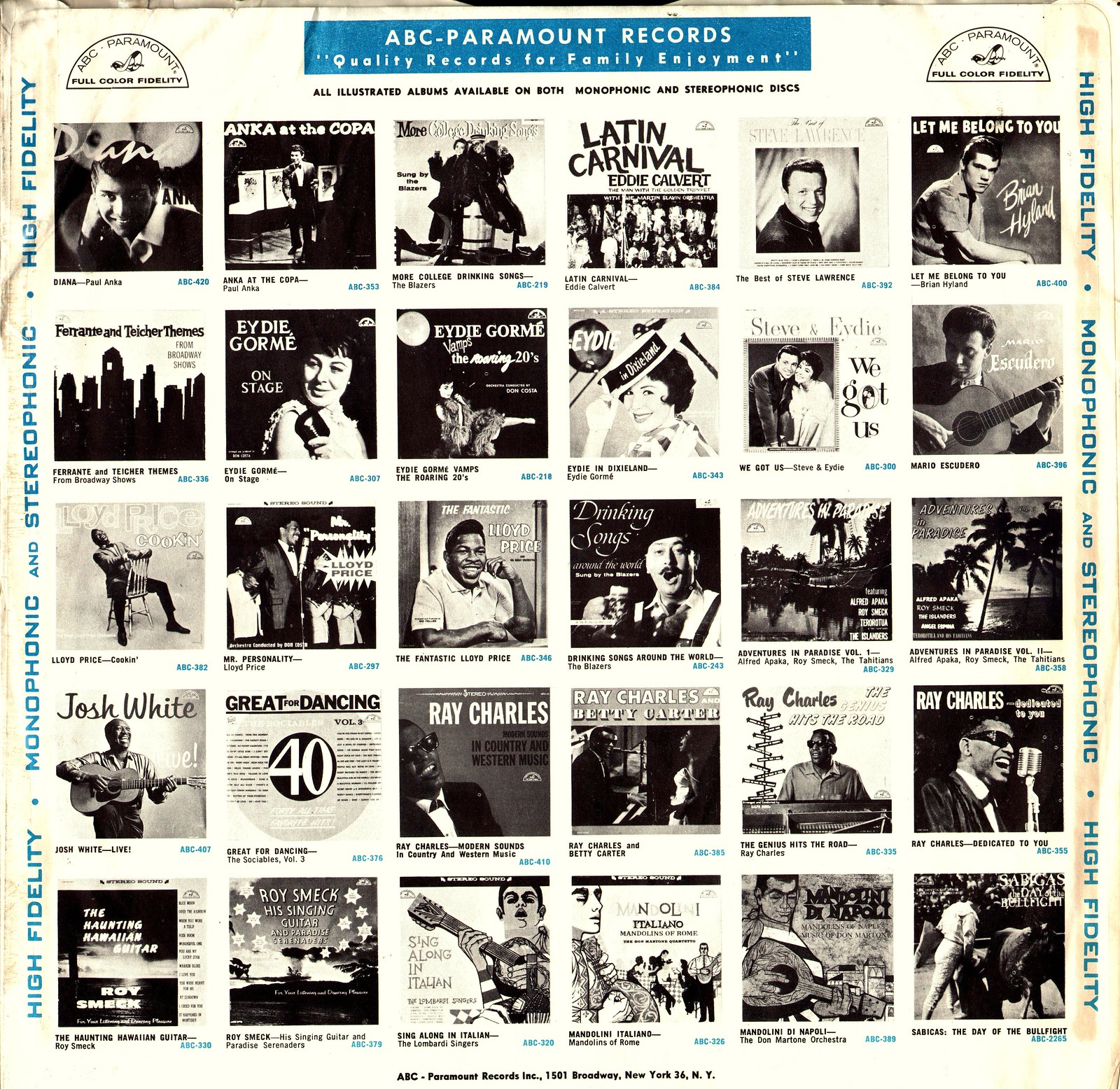This vintage advertising poster for ABC Paramount Records showcases a collection of albums from the record company's diverse catalog. Prominently displayed at the top in blue lettering, the ABC Paramount Records logo is accompanied by the slogan, "Quality Records for Family Enjoyment." The poster is predominantly black and white, with a grid arrangement featuring approximately thirty album covers from well-known artists such as Ray Charles, Edie Gourmet, Paul Anka, Lloyd Price, and Josh White, among others. Each album cover is detailed in monochrome, emphasizing the historical feel of the poster. On either side, the edges are lined with blue text that reads "High Fidelity Monophonic and Stereophonic," highlighting the audio quality available in both formats. Additional black text at the bottom margin provides the company's address: ABC Paramount Records, Inc., 1591 Broadway, New York, 34 NY. The poster, likely from the 1950s, serves as a nostalgic advertisement for the wide array of albums offered by ABC Paramount Records.